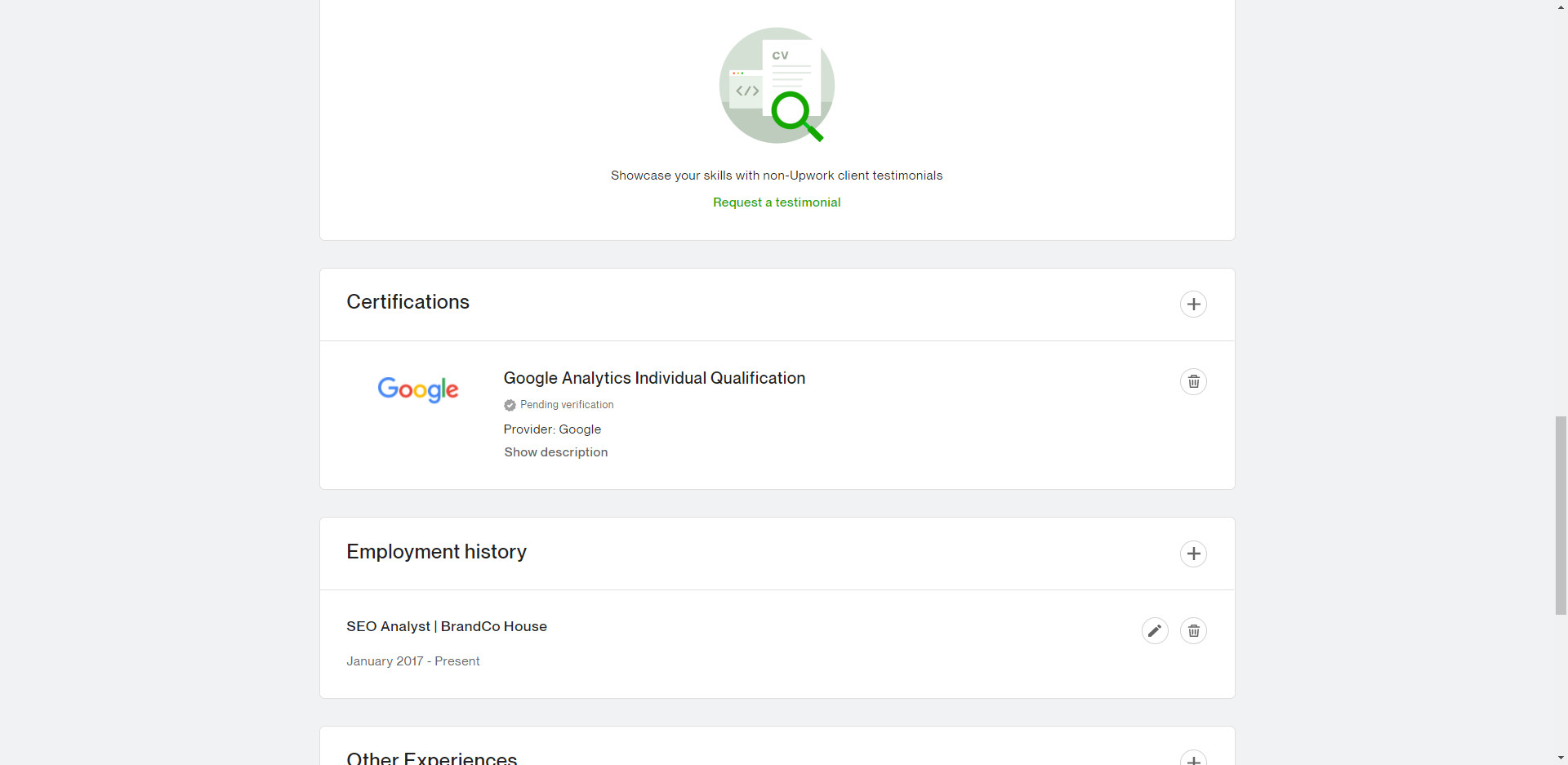The image showcases an organized and detailed profile page, likely from a professional network or freelance platform, with a clean design against a gray background. The layout includes multiple white sections arranged vertically.

At the top of the page, there's a section featuring a small circular avatar with "CV" written on it, set against a backdrop resembling a document. Adjacent to this is a graphical illustration containing a green magnifying glass icon, suggesting a focus on search or investigation.

Directly below this image, the text in bold black reads, "Showcase your skills with non-Upwork client testimonials," followed by a green button labeled, "Request a Testimonial."

The next section titled "Certifications" has a plus symbol on the right side indicating the option to add more. Within this box, the Google logo is prominently displayed alongside text reading, "Google Analytics Individual Qualification, Pending Verification, Provider: Google." To the right of this information is a trash can icon for deleting the certification entry.

Following this, the "Employment History" section also features a plus symbol on the right for adding new entries. It lists a position: "CEO Analyst at Brand Co-House" with the dates "January 2017 - Present." To the right of this entry are two circular icons: one with a pencil for editing and another representing a trash can for deletion.

The final section titled "Other Experiences" includes another plus symbol within a circle on the right side, suggesting the option to add additional experiences.

The overall design is sleek, functional, and emphasizes user interaction with editable and expandable components.